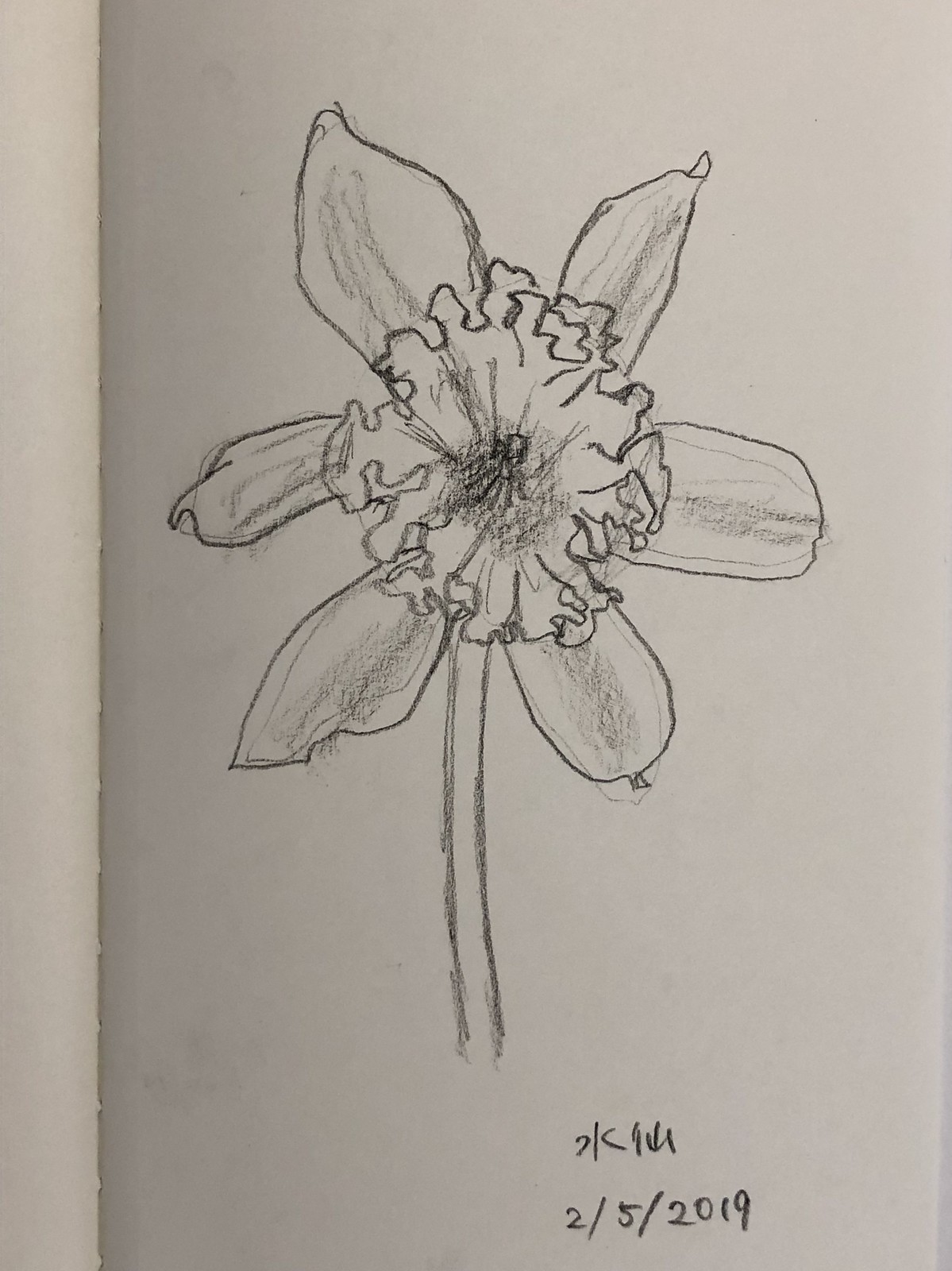This detailed pencil sketch, dated 2-5-2019, features a meticulously drawn flower that resembles a daffodil. Rendered in black and white on a piece of possibly off-white sketchbook paper, the drawing showcases six large petals encircling the main flower, which has ruffled edges arranged in a circular form. The flower's stem extends gracefully downward from the center. The artist's initials are inscribed above the date in the lower right corner, though they are difficult to decipher, possibly containing a "K" or a "U". The sketch, occupying the entire page, captures the delicate details of the flower, including squiggly lines and a small dark spot in the center, creating a striking and elegant portrayal.